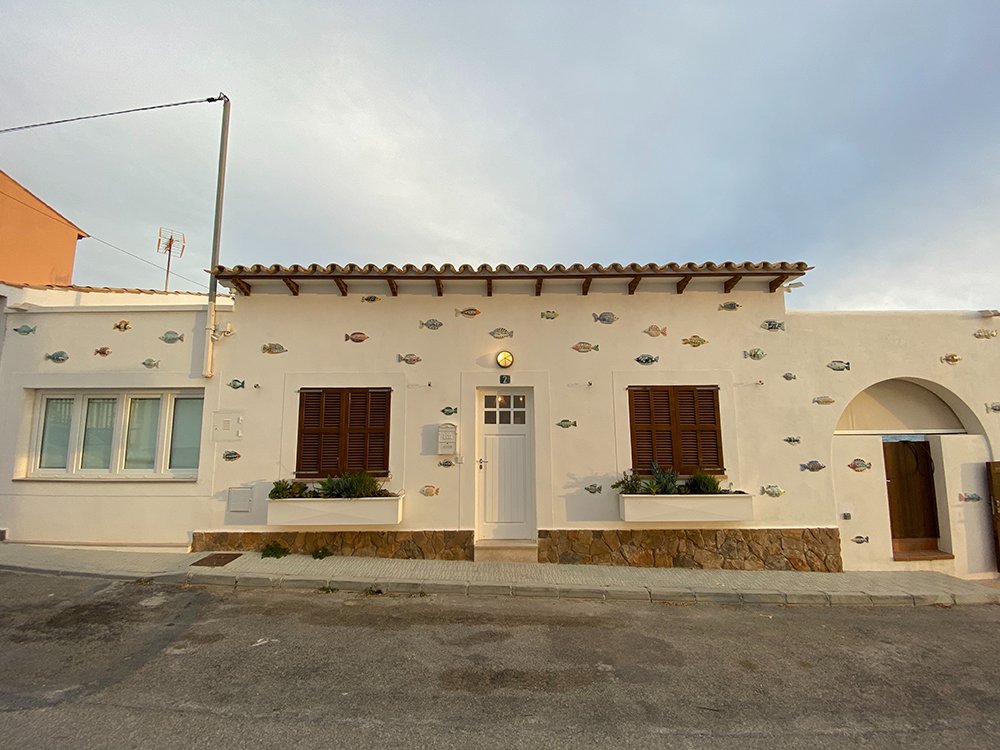This image captures a one-story, light cream-colored building with a flat, rectangular facade. The building features a central white door with small windows, flanked by brown wooden shutters covering the windows on either side. Beneath each window are box planters filled with vibrant plants and flowers. The walls are decorated with an assortment of colorful fish decorations, each unique in size and design, facing various directions. This whimsical fish theme gives the impression that the building might be related to fishing, possibly a business selling fishing equipment or bait, though it could also belong to an enthusiastic fish lover. The structure stands on a slightly sloped gray sidewalk leading to a paved street, which shows signs of patchwork. Above, the sky is mostly cloudy with glimpses of blue, suggesting an overcast day.